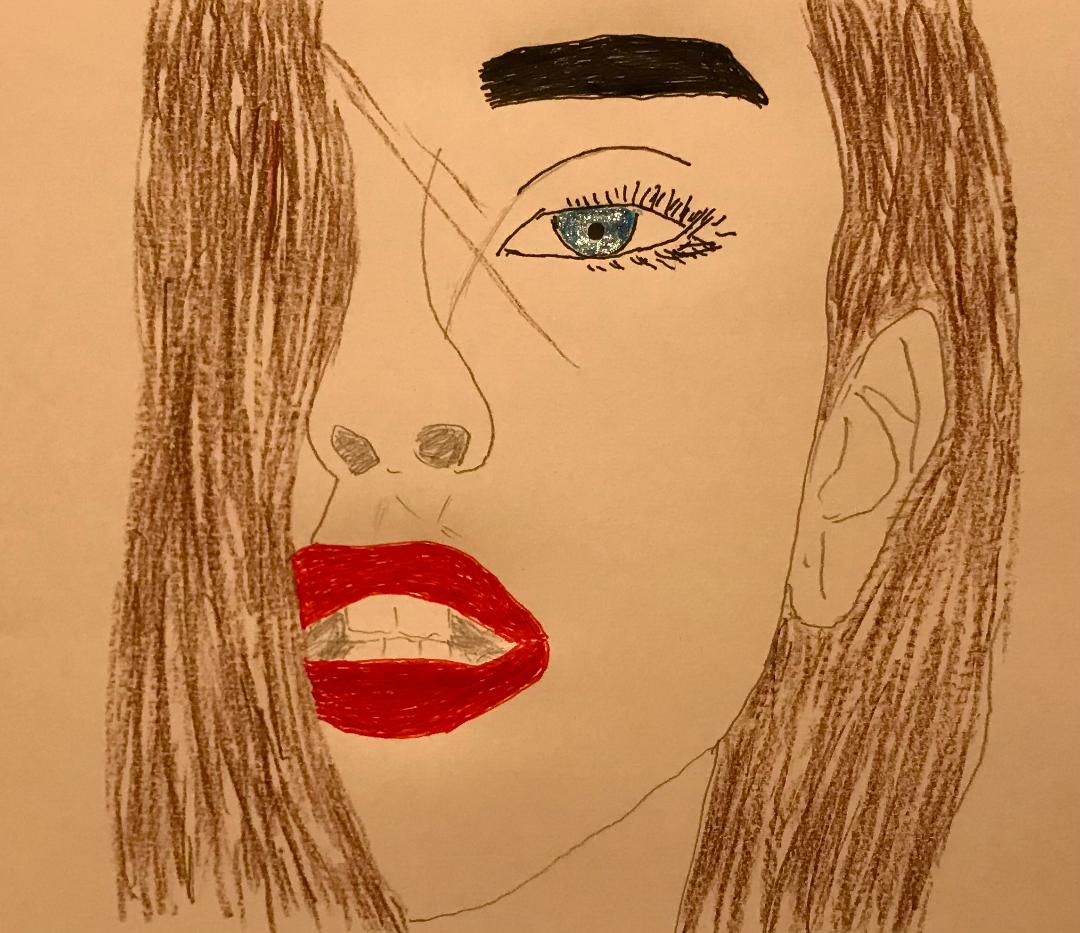This is a detailed drawing of a woman on peach-colored paper, executed with crayon and pencil. She has long, straight brown hair that cascades over one of her eyes, partially obscuring her face. The visible eyebrow is thick and black, complementing her detailed blue eyes adorned with noticeable eyelashes. Her nose is finely drawn, with clearly defined nostrils. The woman has vibrant red lips, slightly parted to reveal two upper teeth and three lower teeth. Her other ear is partially visible as the hair on that side is neatly tucked behind it.